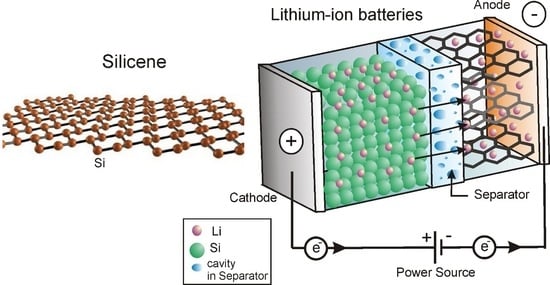The image features a detailed, colorized 3D diagram of a lithium-ion battery, serving as an educational tool for understanding battery operation. Central to the diagram is a vividly illustrated internal structure of the battery, showing various components and their functions.

On the left-hand side is the silicene section, depicted with brown orbs connected by black lines, representing Si. The right side illustrates the lithium-ion battery component, highlighted with numerous green orbs, indicative of Li, separated by a blue wall labeled as the separator, which features blue dots. This separator divides the anode on the right, characterized by hexagon-like black lines with pinkish-orange dots, from the cathode on the left.

The diagram also includes directional arrows labeled 'E', moving from left to right, indicating electron flow. The top corners of the image denote the polarity with a plus sign on the left and a minus sign on the right, clearly marking the cathode and anode areas, respectively. Additional annotations clarify various elements with a legend: pink orbs (Li), green orbs (Si), and blue orbs (representing cavity and separator). The entire setup demonstrates the alignment of positive to negative terminals, essential for establishing the power source in the battery system.